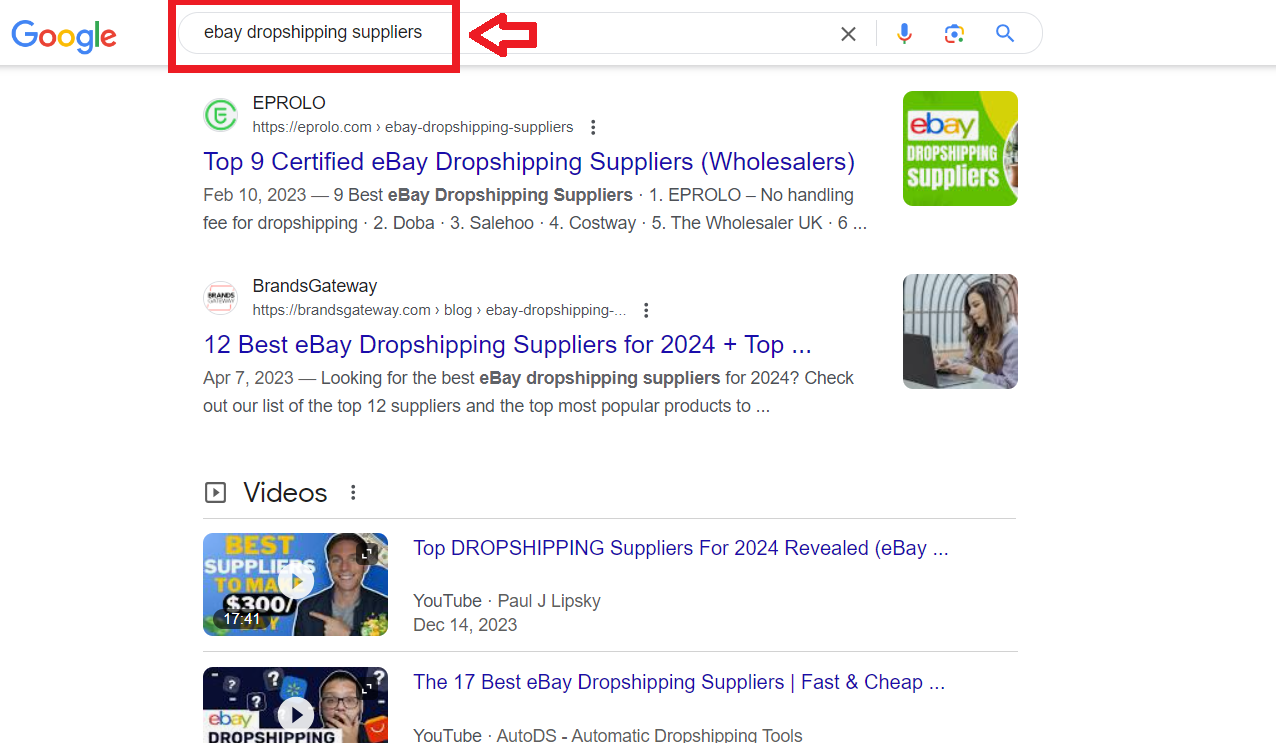This rectangular landscape image is a screenshot capturing a Google search results page viewed on either a laptop or a desktop. The interface is characterized by a predominantly white background, lacking any visible borders. At the top, we see the standard Google header row, underlined by a somewhat thick, light gray line running horizontally across the entire width of the image.

In the top-left corner, Google's multicolored logo is prominently displayed. Adjacent to it, occupying the center of the header row, is a rectangular search bar containing the text "eBay dropshipping suppliers." This text is highlighted by an overlaid, cherry red colored box, which includes a bit of cushioning around the edges, emphasizing the search query. Pointing towards this box from the right is a red-bordered arrow with a white interior.

To the right of the search bar are the standard icons: a small "X," a colored microphone icon, an image icon, and a blue search icon represented by a magnifying glass.

Below the gray bar are the results of the search query, with a detailed layout that provides room for side margins on the left and right. Here are the descriptions of the visible search results:

1. **First Search Result:**
   - **Title:** EPROLO (displayed in all caps)
   - **URL:** An HTTP address related to EPROLO
   - **Logo:** A green circular icon with a line green outline and an "E" in the middle
   - **Snippet Title:** "Top 9 Certified eBay Dropshipping Suppliers (Wholesalers)" in strong blue font
   - **Snippet Text:** Detailed text in gray font, beginning with "Feb 10, 2023 – 9 Best eBay Dropshipping Suppliers," followed by an extended description spanning two lines.
   - **Image:** A square image with a lime green background, featuring the word "eBay" in its standard font, and "Dropshipping Suppliers" below it in white. This image seems to be related to EPROLO.

2. **Second Search Result:**
   - **Title:** Brands Gateway (displayed with capitalized "B" and "G")
   - **URL:** The HTTPS address of Brands Gateway
   - **Logo:** A small, hard-to-read, white circular logo with text
   - **Snippet Title:** "12 Best eBay Dropshipping Suppliers for 2024 + Top..." in blue font
   - **Snippet Text:** Detailed content in smaller gray font, starting with "APR 7, 2023 – Looking for the best," continuing for two lines.
   - **Image:** A square image with rounded corners showing a woman sitting at a laptop, facing left, the laptop positioned in the lower left corner.

Below these main search results is a section dedicated to videos:

- **Videos Section:**
  - Title: "Videos" in gray, with three vertical dots aligned to the right and a box with a right-facing arrowhead to the left.
  - **First Video Result:**
    - Thumbnail: A landscape rectangle with curved corners containing an image of a man pointing over his right shoulder towards some text. A white circle with a right-pointing arrowhead appears on the thumbnail.
    - Duration: Timestamp in the lower left corner shows "17:41.”
    - Video Title: "Top Dropshipping Suppliers for 2024 Revealed (eBay...)" in blue text.
    - Source: "YouTube – Paul J Lipski," with a date of "DEC 14, 2023.”
  - **Second Video Result (Partially Visible):**
    - Thumbnail: Similar format, showing the top two-thirds of a different man with glasses and dark hair, hand covering his mouth.
    - Title: "The 17 Best eBay Dropshipping Suppliers | Fast and Cheap..." followed by an ampersand.
    - Source: "YouTube – Auto DS – Automatic Dropshipping Tools.”

This image offers a comprehensive view of the Google search results page, highlighting specific elements and providing intricate details about logos, text, images, and layout.